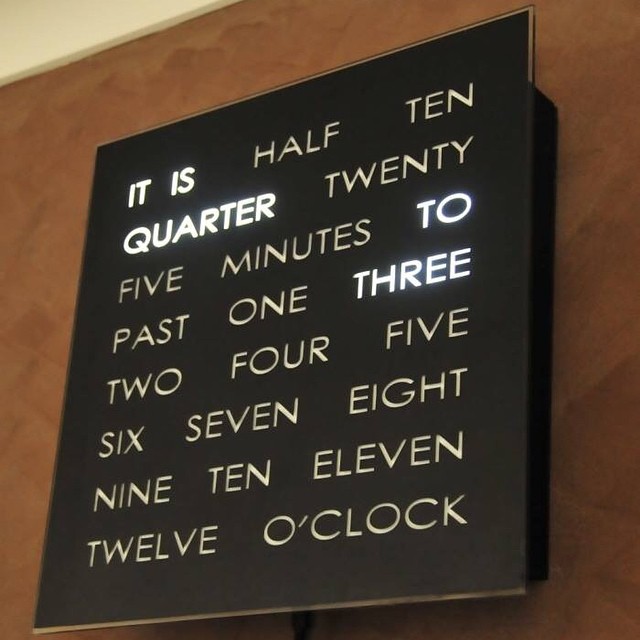The image shows a distinct wall clock with an unusual design, mounted on a two-toned wall where the bottom portion is a smooth, clay-like light brown and the top portion transitions to a whitish color. Positioned centrally on the wall, the clock features a square sign with a black background and numerous words written across eight rows, each containing two to three words. The words displayed on the clock include phrases like "it is half ten quarter twenty five minutes to past one three two four five six seven eight nine ten eleven twelve o'clock." The innovative clock highlights the current time by illuminating specific words. In this instance, the words "it is quarter to three" are glowing, indicating the time. This backlit design cleverly directs the user's attention to the illuminated words to read the current time.